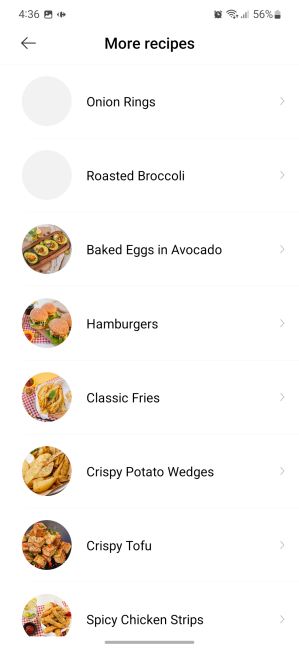This screenshot captures a mobile phone display showcasing various recipes. The interface against a white background features the status bar at the top. On the top left, the time is displayed as "4:36," accompanied by two icons. On the top right, there is a sequence of icons including a battery indicator showing "56%," followed by icons for signal strength, Wi-Fi connectivity, and another symbol.

Central to the screen, below the status bar, is a bolded title "More Recipes." To the left of this title, there is a left-facing arrow indicating a return option to the previous menu. Below the title is a list of recipes, each accompanied by a small image or placeholder.

1. **Onion Rings**: Accompanied by an empty gray circle, which typically would feature a product shot.
2. **Roasted Broccoli**: Similar to the onion rings, this entry has an empty gray circle to its left.
3. **Baked Eggs and Avocado**: Features a thumbnail image showing avocados topped with egg yolk.
4. **Hamburgers**: Includes a thumbnail of a fully-topped burger cut in half.
5. **Classic Fries**: Displays a dish of fries with sauce in a photograph on the left.
6. **Crispy Potato Wedges**: Comes with a thumbnail image of well-cooked potato wedges.
7. **Crispy Tofu**: The picture showcases square pieces of crispy tofu.
8. **Spicy Chicken Strips**: Illustrated with a photograph of chicken strips accompanied by a small dipping sauce bowl.

Overall, the screenshot conveys a structured layout of enticing food recipes, enhanced by corresponding images or placeholders.